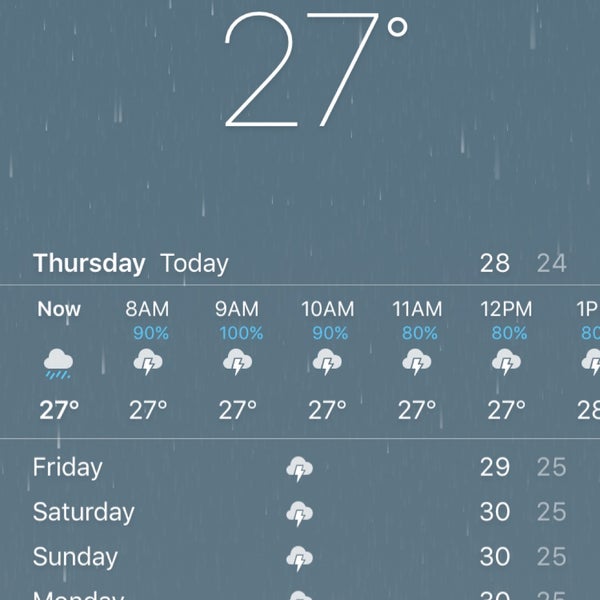A screenshot of the weather forecast displays current conditions and upcoming weather for the next several hours. The current temperature is 27 degrees with rain. The detailed forecast is as follows: 

- 8:00 AM: 90% chance of showers
- 9:00 AM: 100% chance of thunderstorms
- 11:00 AM: 80% chance of thunderstorms
- 12:00 PM: 80% chance of thunderstorms
- 1:00 PM: Continued thunderstorms

The forecast is presented on a grey background with white text, accompanied by small cloud icons to represent the thunderstorms. The days mentioned, Friday, Saturday, and Sunday, also predict thunderstorms.